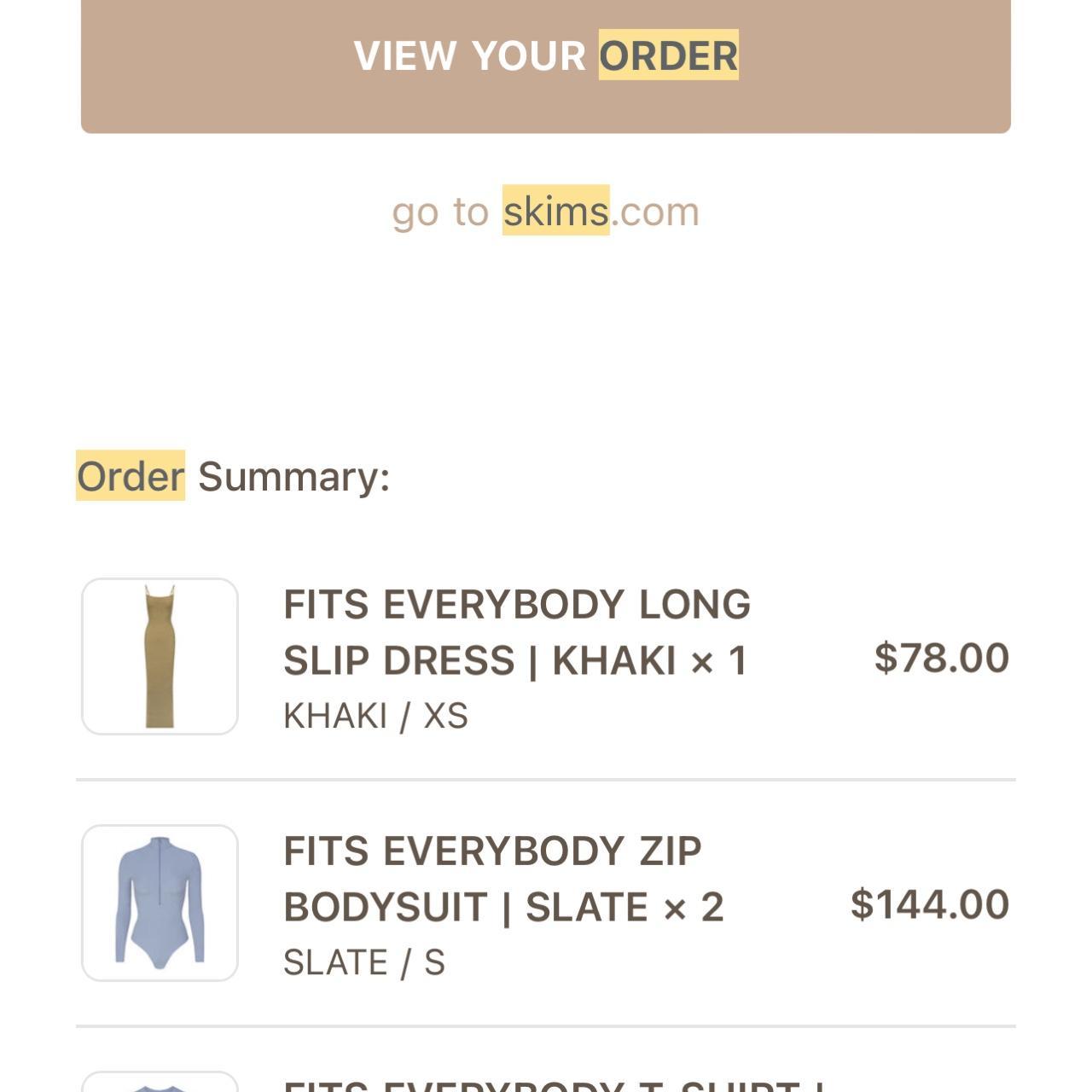This image features a screenshot of a web page from the Skims website. The page has a soft nude color that spans from left to right. At the top, there's a highlighted "Order" button in yellow with the text "View your" in bold, white lettering. Below it, there's the text "Go to skims.com," with "skims" highlighted. 

The page also displays an "Order Summary" section with several items listed. The first item is a "Fits Everybody Long Slip Dress" in khaki, ordered in size extra small, priced at $78. To the left, there's a square image of the dress. 

The second item listed is a "Fits Everybody Bodysuit" in slate, with two ordered for a total cost of $144, accompanied by an image of the bodysuit on the left.

Further down, there's a partially visible item, showing the text "Fits Everybody" but cut off, revealing only about an eighth of the text and a small portion of the item on the left. The bottom of the web page is also cut off, hinting that additional information is present but not visible in the current view.